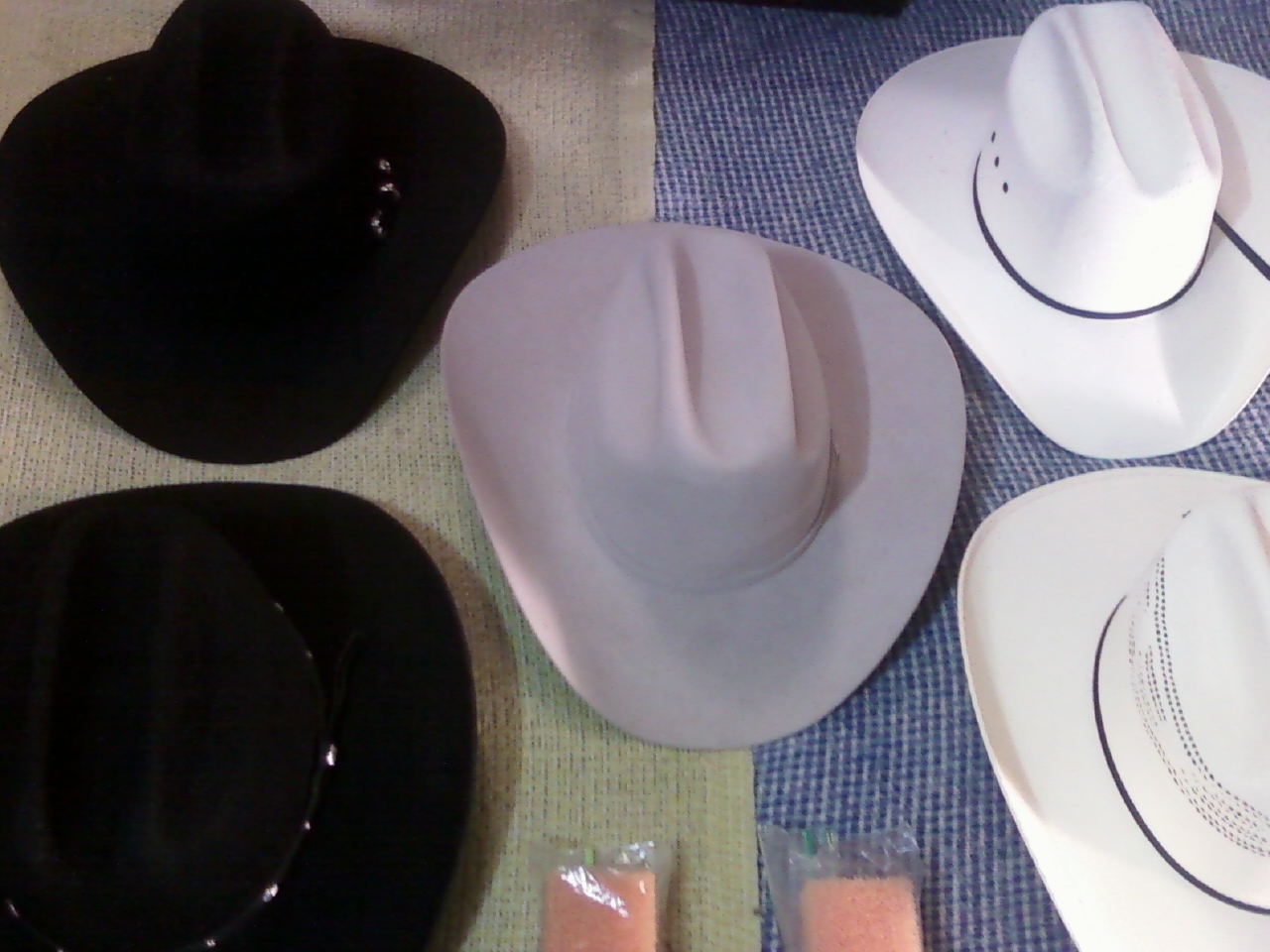This indoor color photograph captures a detailed and organized display of western cowboy hats on a table draped with a tan cloth on the left and a blue cloth on the right. Five hats are prominently laid out: two black hats with black bands studded with silver embellishments on the left, a plain gray hat in the center, and two white hats with wide brims on the right. The white hats feature distinctive ventilation designs–one with three holes and the other with a pattern of holes encircling the crown. Both white hats have a single black string tied near the brim. In the foreground, two woolen scarves are placed under the hats, one in blue and the other in a vanilla color. Additionally, two pink, soap-like items wrapped in plastic are visible at the bottom of the image. The lighting highlights the setup, creating a slightly darker tone on the left side and a lighter tone on the right.